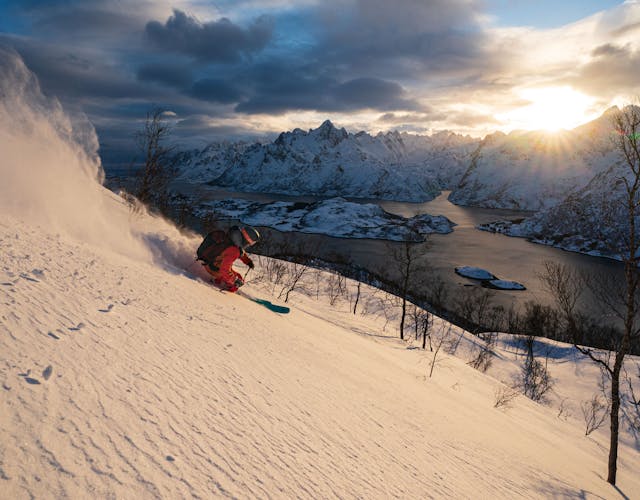This dynamic photo captures a skier, dressed in a striking red coat, paired with a black backpack and helmet, carving gracefully down a snowy hill. Their blue skis are angled towards the right, indicative of their leaning posture as they navigate the moderate slope. The skier is moving fast down the hill, nearing the bottom where the silhouette of bare trees begins to emerge. 

The background is dominated by a rugged, snow-covered mountain range, over which the setting sun casts golden beams, partially obscured by heavy gray clouds. The sun, nestled behind the distant mountains, lights up the scene with a yellowish-white hue from the right side of the picture. Below, a river snakes through the landscape, appearing frozen with a sheen of white ice, and dotted with small, snowy islands. All these elements come together to perfectly frame a moment of swift motion against a breathtaking winter vista.